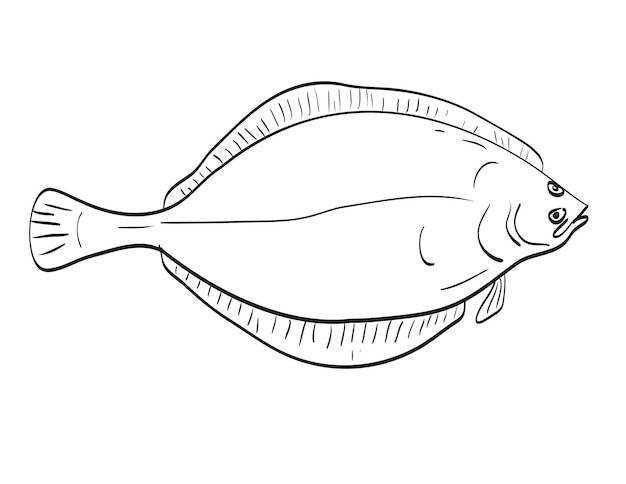The image is a black-and-white, simplistic graphic design of a fish, much like a fish coloring page. The fish is depicted in an outlined sketch against a white background, stretching from the left side to the right side of the image. The fish's body has an oval-like shape with a large stomach area tapering towards a fan-shaped tail on the left. The fish has its mouth open on the right side, revealing two black eyes. The top eye is round with a dark circle in the center, while the lower marking, which might be a gill, also appears prominently. One small fin is visible towards the bottom front, detailed with black lines, and further fins extend along the top and bottom of the fish. The outer edge of the fish is defined with black lines, featuring additional markings along the tail and fins. Overall, the drawing is quite large and detailed considering its simplistic nature.